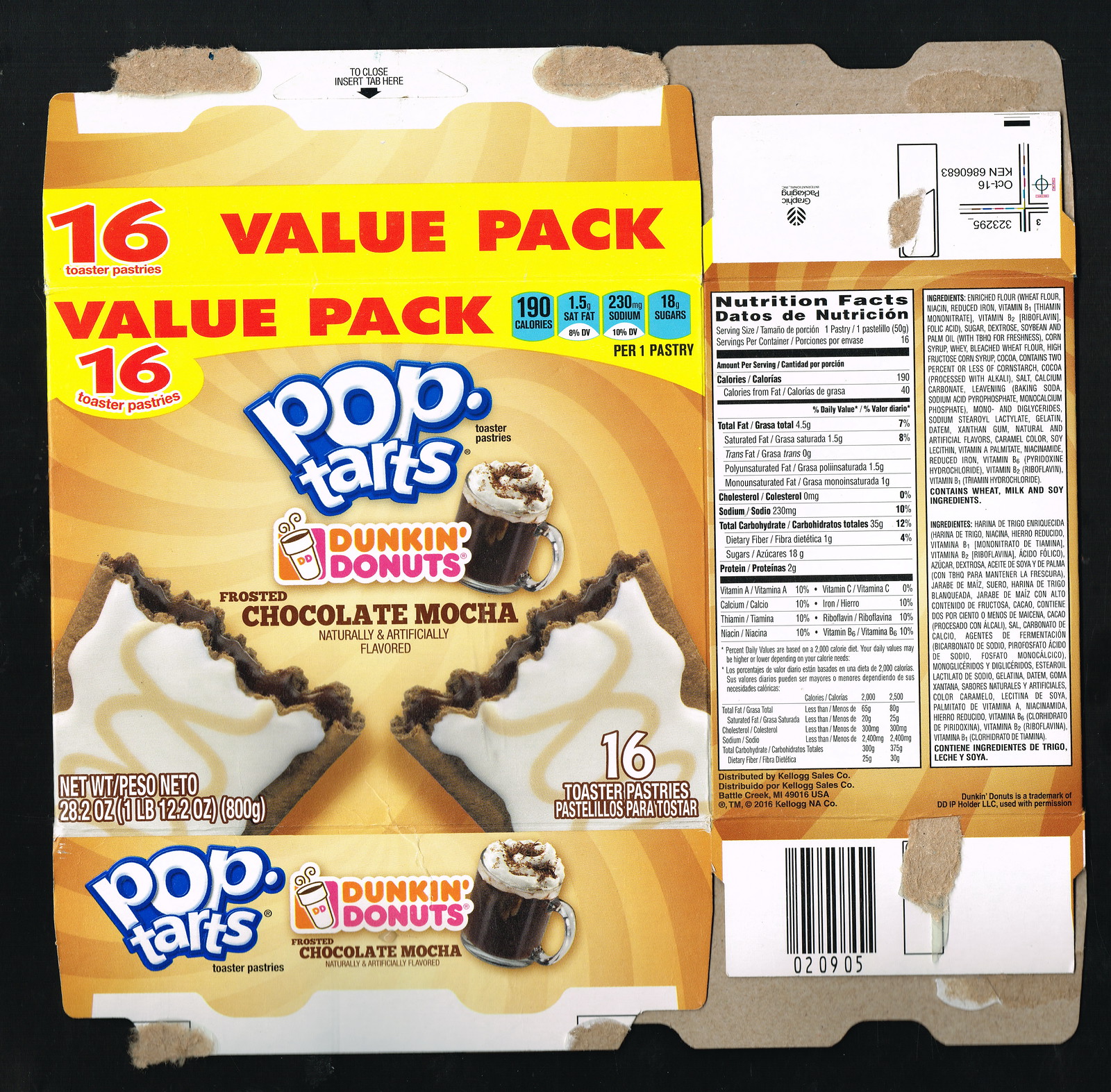A meticulously detailed photograph captures a fully flattened Pop-Tarts box set against a pure black background, enhancing its visibility. The cardboard box, printed in captivating swirls of orange and cinnamon hues, is completely laid out. Positioned on the left-hand side of the image, the top of the box prominently displays "16 Value Pack" in bold yellow text. Below this, nutritional information is organized into neat blue tabs.

Central to the design, 'Pop-Tarts' is emblazoned in large print, accompanied by the recognizable Dunkin' Donuts logo. Adjacent to this is an enticing image of a glass mug filled with a dark liquid presumed to be coffee, adorned with cream and topped with chocolate. 

The bottom section showcases the featured product, with two richly colored Pop-Tarts emerging from each corner. These pastries, covered in white icing and adorned with a caramel-colored helix pattern, emphasize the flavor: Frosted Chocolate Mocha.

Flanking the main section, two vertical panels are visible; one displays detailed nutrition facts on a white background, while the other outlines the list of ingredients, ensuring the consumer is well-informed. This thorough depiction captures every aspect of the box’s design and information in a visually striking manner.